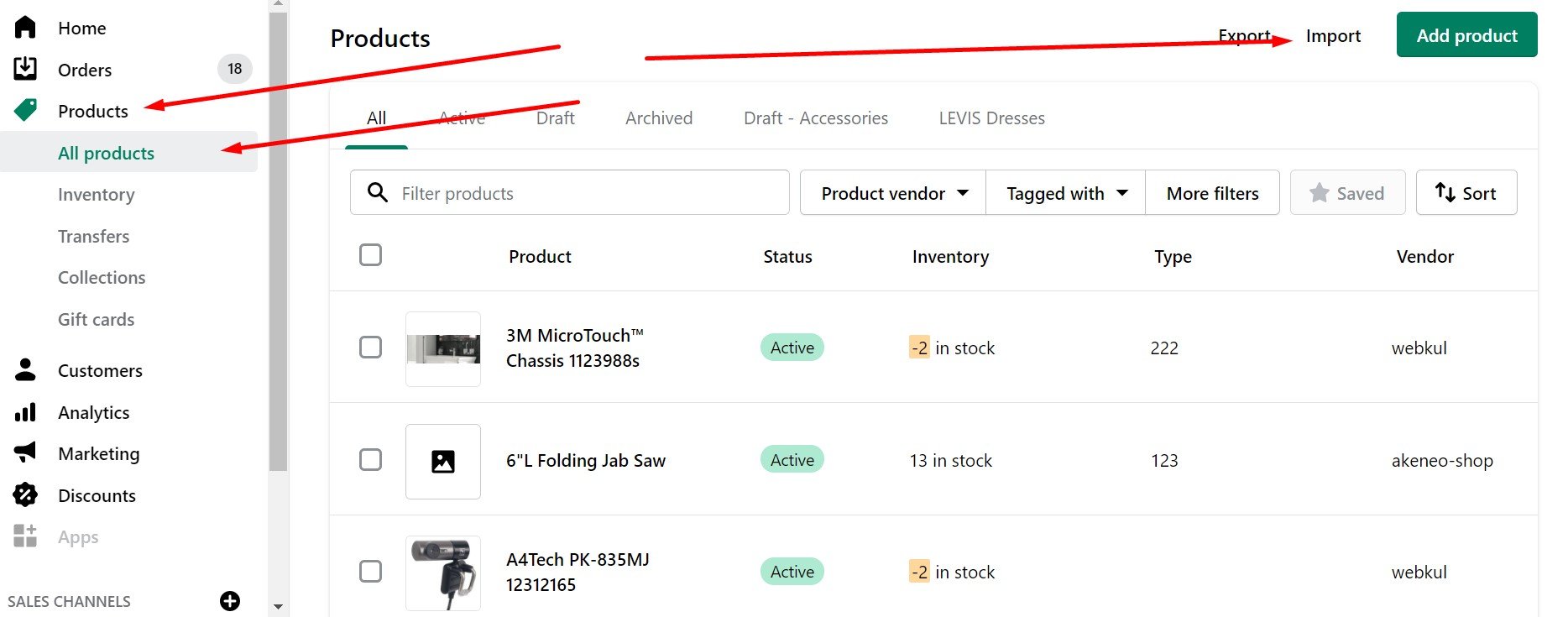The image displays a detailed interface of a product management dashboard. On the left side, there's a vertical gray scroll bar separating a narrow side panel from the main content. 

**Left Panel:**
- The panel header features the word "Home" and "Orders" highlighted in black within a gray circle with the number 18 beside it.
- Below that, "Products" is displayed prominently with a red arrow pointing to it.
- "All Products" is highlighted in green within a gray rectangle, accompanied by another red arrow.
- Subsequent gray text includes "Inputs for Retransfers," "Collections," and "Gift Cards."
- Then in black, "Customers," "Analytics," "Marketing," and "Discounts" are listed.
- "Apps" is presented in gray, followed by "Sales Channel." 
- Adjacent to "Sales Channel," a black circle with a white plus sign is visible.

**Main Content Area:**
- The section is headlined with "Products" in black text, followed by clickable options "Export" and "Import," both noted in black with an associated red arrow.
- A prominent green rectangle with white text reads "Add Product," indicating an option to add new products.
- Underlined in gray, the categories "Active," "Graph," "Archive," and "Draft-Accessories" are listed, alongside "LEVIS Addresses."
- A search box labeled "Filter Products" is featured with a black arrow pointing towards it.
- Adjacent to the search box, options in black text include "Product Vendor," "Tagged with," and "More Filters" with an adjacent gray "Saved" indicator.
- The "Sort" option, displaying up and down black arrows, allows sorting functionality.
- Various filter headings include "Product Status," "Inventory," "Type," and "Vendor."

**Product Listings:**
- Vendors listed include names like "WebCool," "Akeem Yo Shop," and "WebCool" again, indicating the availability of multiple products from various vendors.
- Product types depicted include identifier codes like "222123."
- Inventory counts show "-2 in Stock," "13 in Stock," and "-2 in Stock."
- Product status across the dashboard lists as "Active."
- Products featured include items such as "3M MicroTouch 6-inch L Folding Jabsaw" and "A4Tech PK-835MJ123" with identifiers like "12165."

The image provides a comprehensive view of the options and functionalities available for managing a diverse inventory, clearly highlighting important labels, actionable buttons, and distinctly categorized sections.